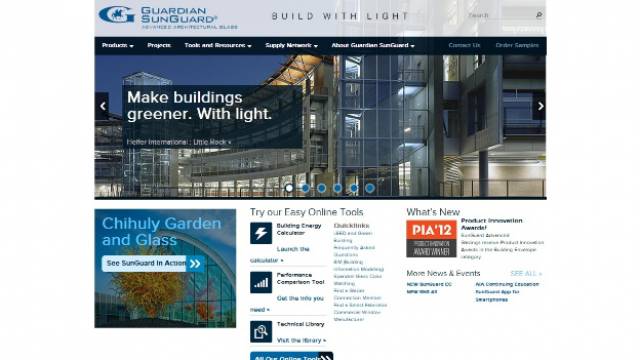A webpage screenshot from Guardian Sun Guard, a company specializing in advanced glass features for buildings, prominently displays their tagline "Build with Light." The main header encourages making buildings greener by harnessing light effectively. Although the detailed text content isn't readable, the imagery and headers suggest a focus on various types of glass films designed to regulate light for businesses and offices, enhancing energy efficiency and sustainability. A smaller feature on the left highlights the "Chihuly Garden and Glass" installation, possibly indicating a collaboration or display of the renowned glass artist’s work within one of their projects. In the center of the page, tools such as the "Building Energy Calculator" are offered, emphasizing Guardian Sun Guard's commitment to sustainable building practices through innovative glass solutions.